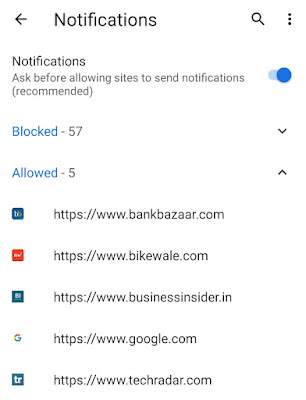The image is a screen capture of a browser's notification settings page. 

At the top, there is a back arrow pointing to the left, indicating the previous page. Adjacent to it, the word "Notifications" is displayed prominently, suggesting that the current section is dedicated to notification preferences. To the right of the title, there is a magnifying glass icon for searching, followed by three vertical dots which open a drop-down menu with additional options.

Below this header, there is a section titled "Notifications." The option "Ask before allowing sites to send notifications" is displayed with a blue toggle switch beside it, indicating that this feature is currently turned on. The text "Recommended" appears in parentheses underneath to suggest this setting is advised.

The main content of the screen shows two categories: "Block" and "Allow." 

- Under "Block," it displays a summary "Block-57" alongside a drop-down arrow. This implies there are 57 websites that have been blocked from sending notifications.
- Under "Allow," it lists "Allowed-5," and this section is already expanded showing the URLs of websites permitted to send notifications: 
  - https://www.bankbazaar.com
  - https://www.bikewhale.com
  - https://www.businessinsider.in
  - www.google.com
  - www.techradar.com

Clicking the up arrow next to "Allowed-5" would minimize this list.